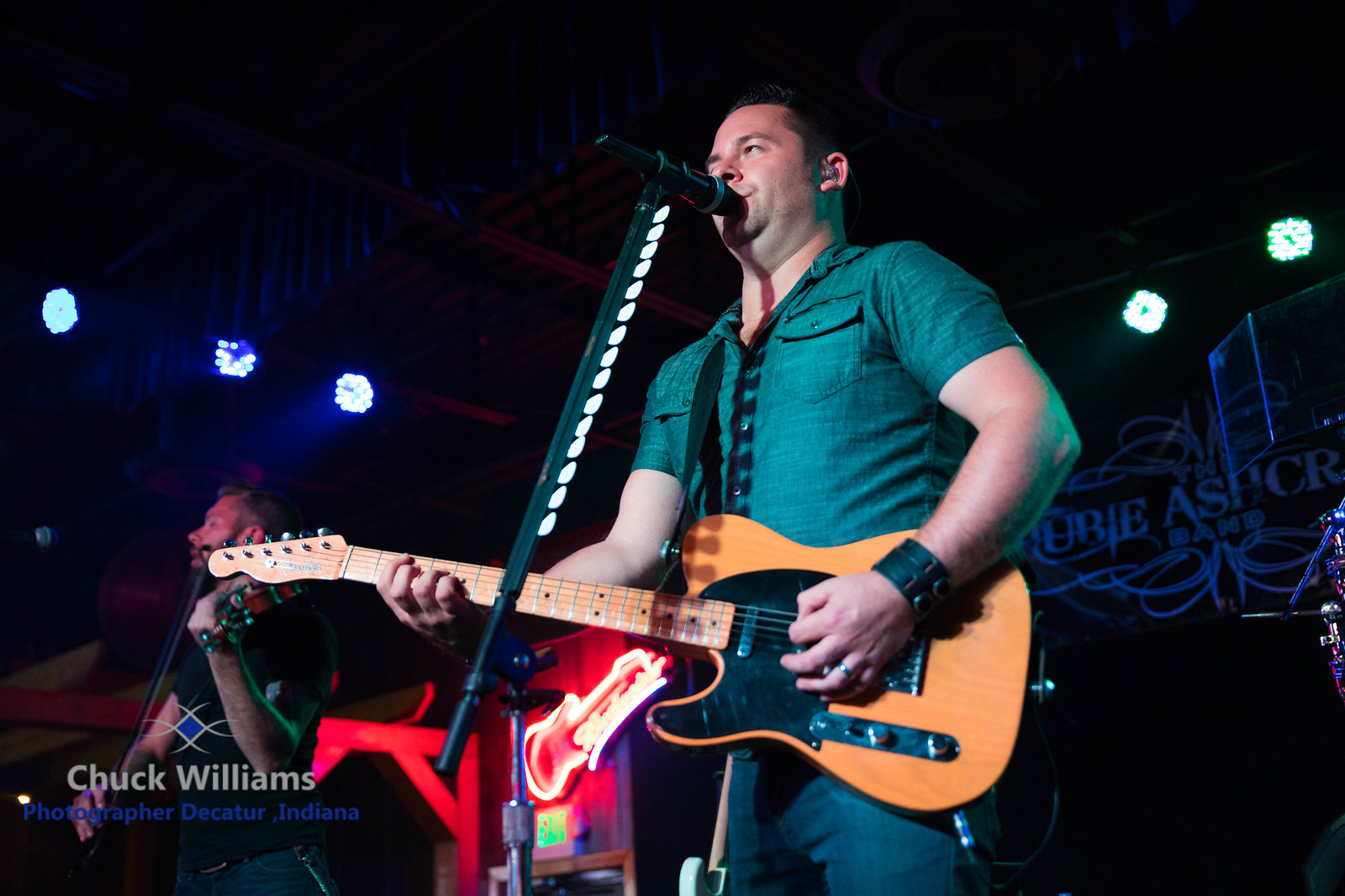In a dark concert setting, illuminated by several high lights, a male singer takes center stage, strumming an orange and black left-handed electric guitar. He wears a green short-sleeve shirt with front pockets and blue jeans. Black leather bracelets and a ring adorn his wrists and fingers, while an array of guitar picks are attached to his microphone stand, which is raised almost to his lips as he sings. Behind him, a partially visible red sign hints at "URIE Ashcroft," suggesting the band or venue's name. To his right, another musician plays the violin, positioning it skillfully against his neck with the bow in his right hand. Both performers are highlighted by bright spotlights in the midst of a largely dark background. The image credits below identify Chuck Williams, a photographer from Decatur, Indiana.